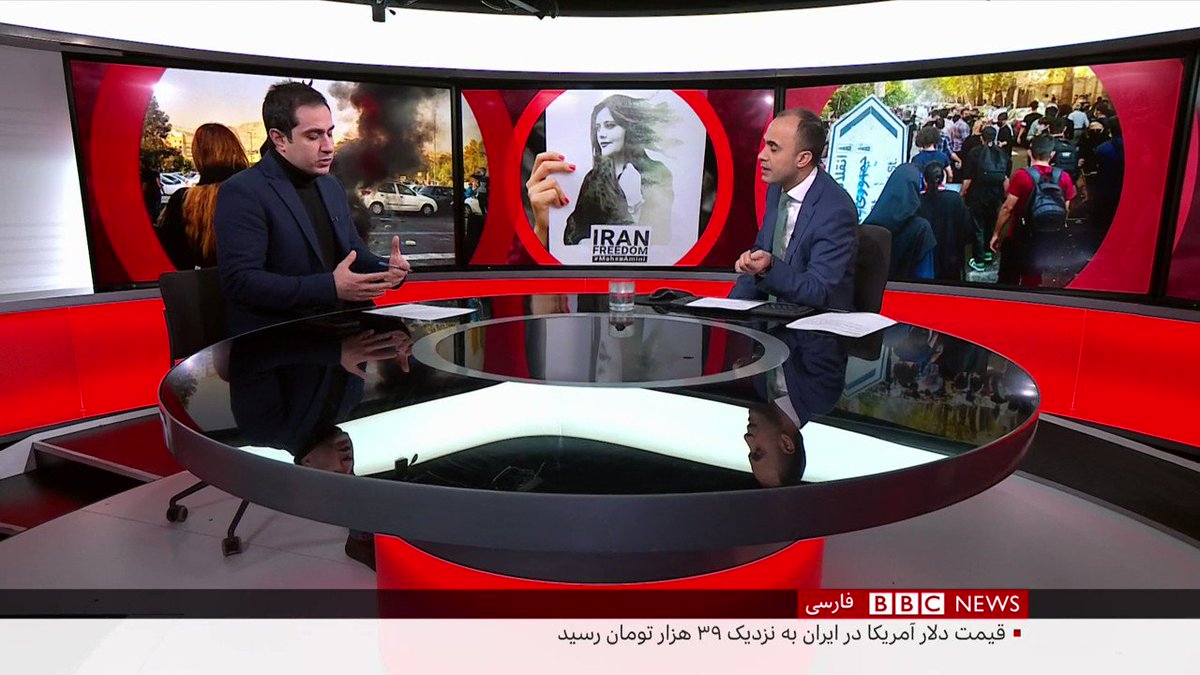This image, evidently from a BBC News broadcast, features two Caucasian men seated at a glossy, reflective black circular table. One man is attired in a blue suit with a white button-up shirt and tie, while the other sports a black suit jacket and turtleneck. Behind them, on large display screens, are three vivid images related to protests. In the center of these images, a woman holds a sign reading "Iran Freedom." To the left is an image of a car engulfed in flames, and to the right, a crowd gathered in protest. The BBC News logo is prominently displayed in red and white, and there is text below it that appears to be in Arabic script.